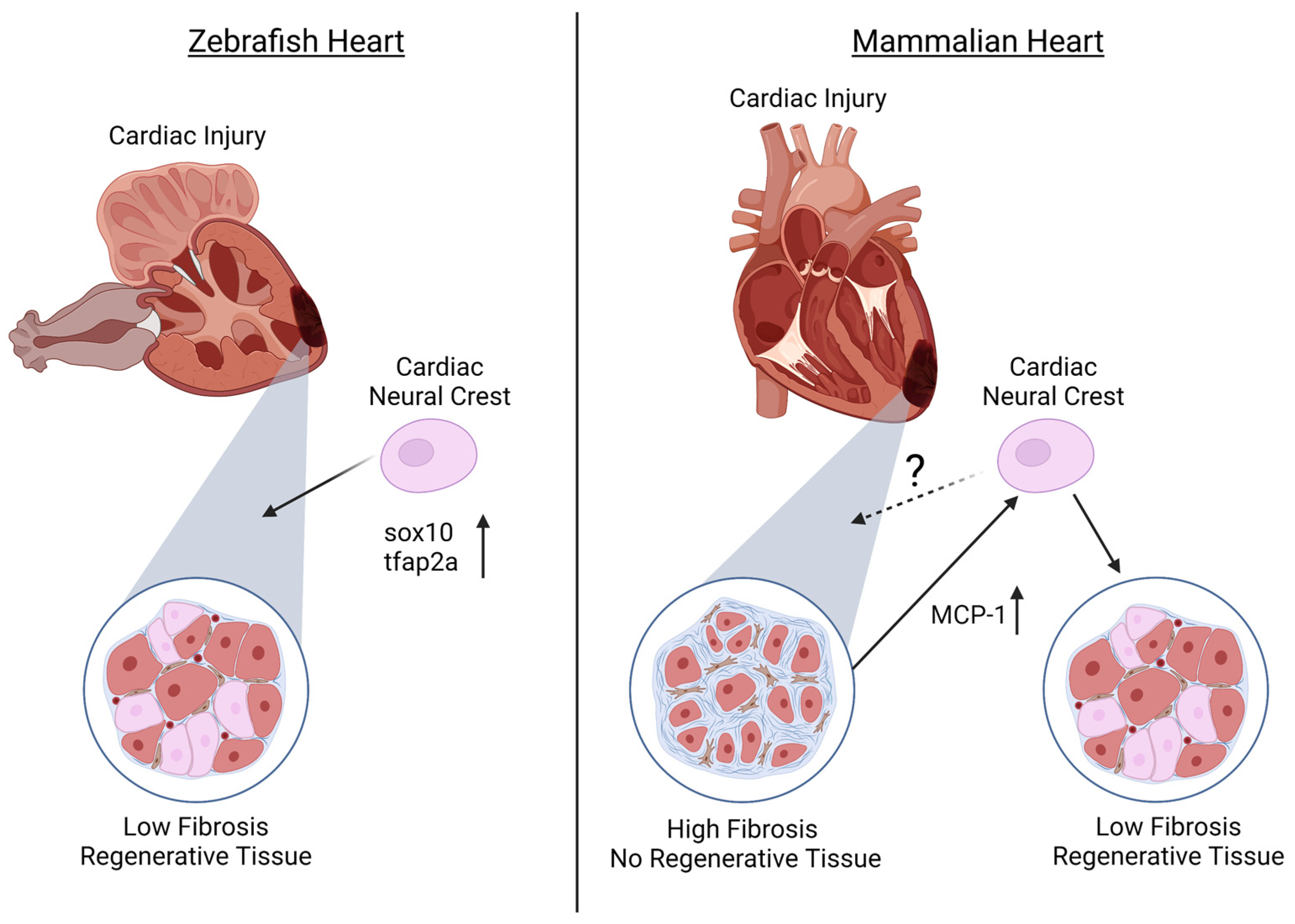The image is a comparative scientific diagram of a zebrafish heart and a mammalian heart, typically seen in a medical or educational setting. On the left side, the zebrafish heart is depicted, characterized by a unique appearance that somewhat resembles a fish or skeleton. The diagram highlights its low fibrosis and regenerative tissue capabilities after cardiac injury, showing detailed anatomical features such as blood vessels and darker regions distinct from the mammalian heart.

On the right side, the mammalian heart is displayed, resembling a typical human heart. The image focuses on the high fibrosis and lack of regenerative tissue following cardiac injury, providing a stark contrast to the zebrafish heart. Both hearts are presented in reddish-pink hues with numerous blood vessels. Central to the diagram is the annotation of the cardiac neural crest, marked by pink circles and arrows, which points out specific tissue structures and differences in fibrotic response. This detailed comparison underscores the divergence in cardiac injury responses and healing potentials between zebrafish and mammals.